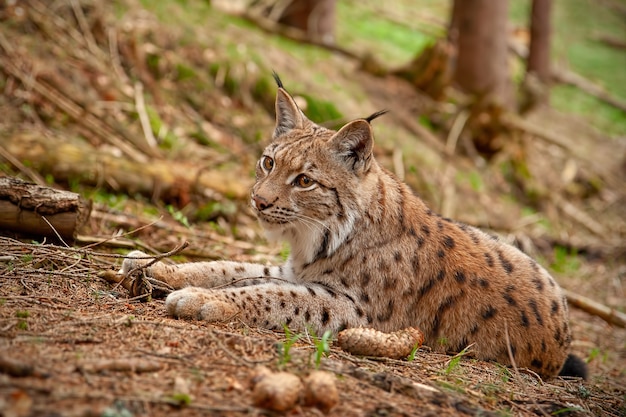This horizontal outdoor photograph captures a young bobcat resting on a forest floor covered with pine needles, grass, and twigs. The bobcat, with its orangey-tan fur accented by black spots and stripes, is presented in clear detail in the foreground, while the background transitions to a blurred mix of trees, greenery, and tree stumps. The animal is positioned facing the left side of the frame, with its front paws stretched out and its gaze directed towards the upper left. Distinctive features include black tufts atop its ears, orange eyes, and lighter-colored fur on its legs. Surrounding the bobcat, the ground is scattered with pine cones and logs, enhancing the woodland atmosphere. The photograph accentuates the serene and solemn demeanor of the solitary feline in its natural habitat.